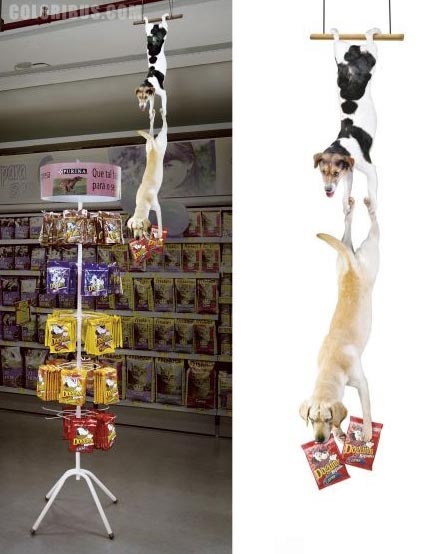The image depicts the interior of a pet store, showcasing a vibrant and bustling display. Dominating the scene is a white metal stand adorned with an array of brightly colored dog treat packages in shades of red, yellow, blue, and brown, accompanied by pink signage with Spanish text, including words like "QUE" and "PARA". In the foreground, a whimsical mobile hangs from the ceiling, featuring two dogs in an acrobat-like pose: a smaller, white dog with black spots and a light brown face dangles by its hind legs from a trapeze, while supporting a larger beige and white dog. The larger dog, possibly a Labrador, is reaching out towards the dog treat display, clutching one bag of treats in its mouth and another between its front paws. To the right of this main image, a close-up provides a detailed view of the two dogs and the treats they are holding, emphasizing their playful and intricate arrangement. The backdrop of the scene includes a white ceiling and a multi-tiered display case filled with additional pet treats, contributing to the inviting and energetic atmosphere of the store.